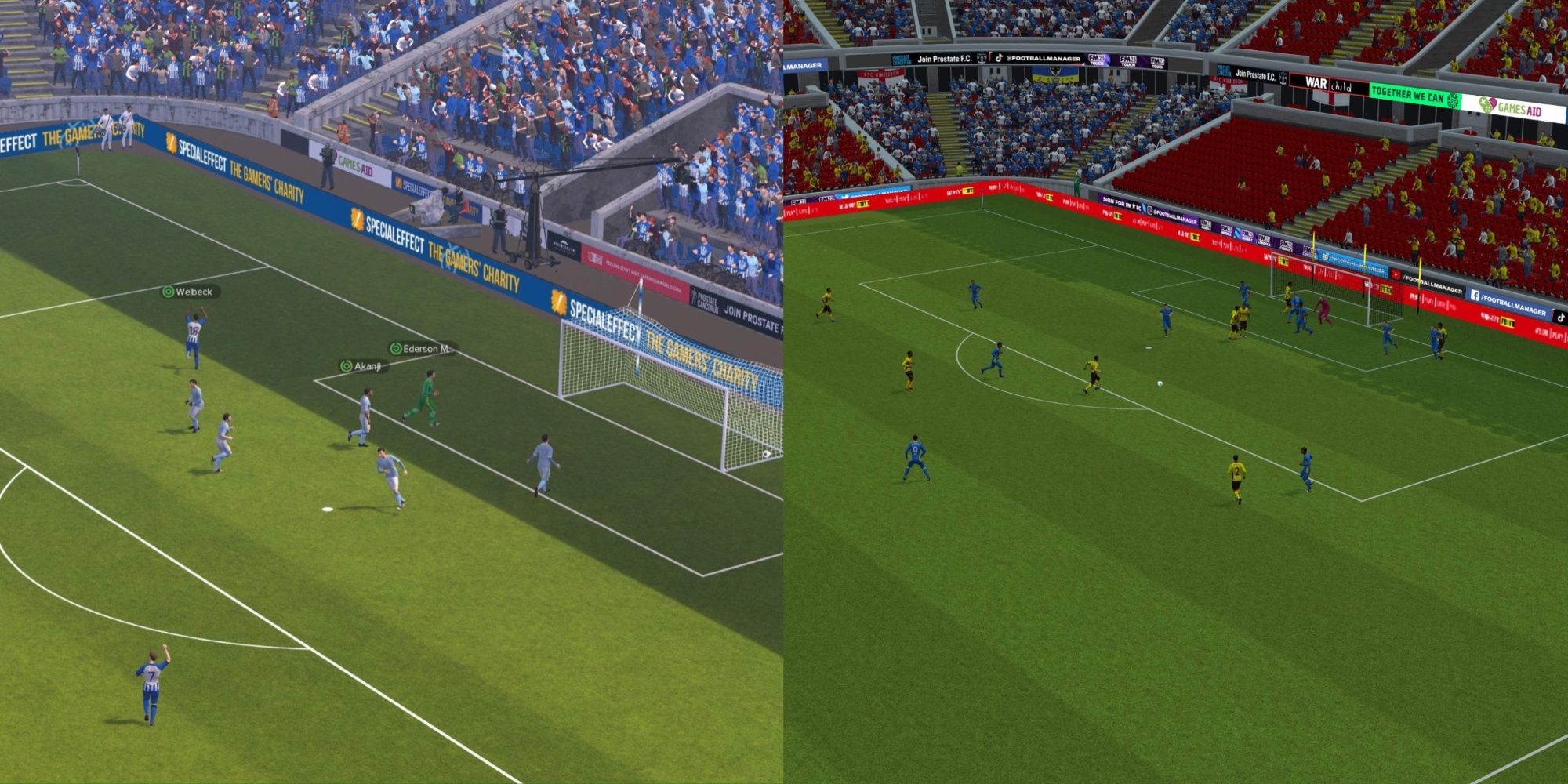This rectangular image is divided into two sections, each depicting a scene from a soccer video game in an aerial, computer-generated view. On the left, a more zoomed-in shot features players dressed in blue and white near one of the goals, with the soccer ball situated inside the net. Fans fill the grandstands in the background, predominantly dressed in royal blue. A blue, white, and yellow banner encircles the field's border. The right side shows a slightly zoomed-out view of a different segment of the field. Here, players are wearing different colored uniforms, including blue, yellow, and black, and the ball is not in the goal. The grandstands are visible but appear to contain fewer spectators, with seats in red. Both sections emphasize vibrant green turf and provide a detailed, immersive look at the in-game soccer action from an elevated perspective.